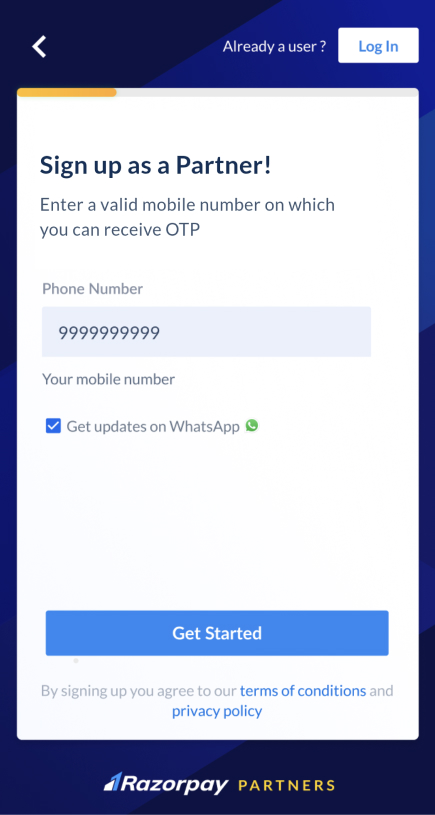This digital image showcases the Razorpay registration interface. At the top, a prompt reads "Already a user?" followed by a question mark. Adjacent to this prompt, there is a "Login" button. Below that, the page offers an option to "Sign up as a partner."

The main section of the image features a text field labeled "Enter a valid mobile number on which you can receive OTP." Here, a sample mobile number, "9999999999," is pre-filled. Underneath this, another label reads, "Your mobile number."

An option to "Get updates on WhatsApp" is displayed with a checked checkbox to its left, indicating the user's consent to receive updates via WhatsApp.

At the bottom of the interface, a prominent blue "Get Started" button invites the user to proceed. Beneath this button, a disclaimer states, "By signing up you agree to our Terms of Conditions and Privacy Policy." Both "Terms of Conditions" and "Privacy Policy" are clickable links, allowing the user to review the terms and policies.